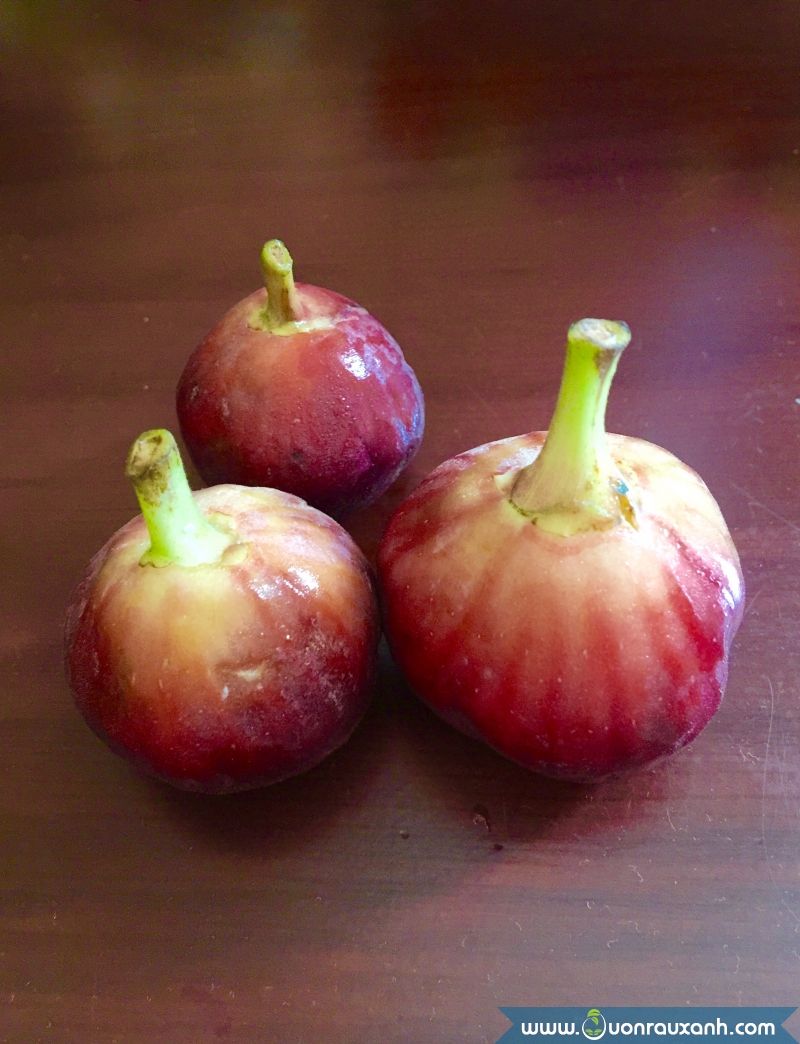In the photo, there are three mature figs exhibiting a rich gradient color from beet red at their bases to a creamy hue nearer their greenish stems. The figs, varying slightly in size, are arranged in a triangle on a scratched and worn wooden table, possibly made of mahogany or dark walnut, with visible wood grain patterns. Each fig has a distinct stem where it’s been cut, with the one on the left being the smallest and the one on the front right the largest. The photo also features the text "www.unrauxanh.com" alongside a small logo of a person inside the letter "U" located in the bottom right corner. The overall composition highlights the aged texture of both the figs and the table surface, illuminated softly by overhead light.